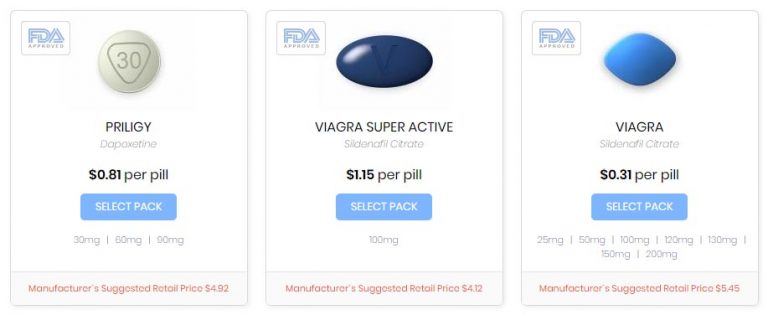The image showcases an array of three FDA-approved medications, each displayed in its own neatly organized box. At the top of each box is the FDA approval symbol, which features blue lines artfully spelling out "FDA" and the word "approved" in black beneath it. To the right of this symbol, a clear image of each respective pill is shown. 

Directly below the images, the name of each medication is prominently displayed and followed by the price per pill. Underneath this information, a blue button labeled "Select Pack" is available for each medication, allowing users to choose their desired quantity or variant. 

Further down, the specific milligrams available for selection are listed. At the very bottom of each box, the manufacturer's suggested retail price (MSRP) is presented in red.

- The first medication is Prilogy, priced at $0.81 per pill. Users can select from three dosage options: 30 mg, 60 mg, or 90 mg.
- The second medication is Viagra Super Active, with a price of $1.15 per pill and a fixed available dosage of 100 mg.
- The third medication is Viagra, which is priced at $0.31 per pill. It offers a wide range of dosages to choose from: 25 mg, 50 mg, 100 mg, 120 mg, 130 mg, 150 mg, and 200 mg.